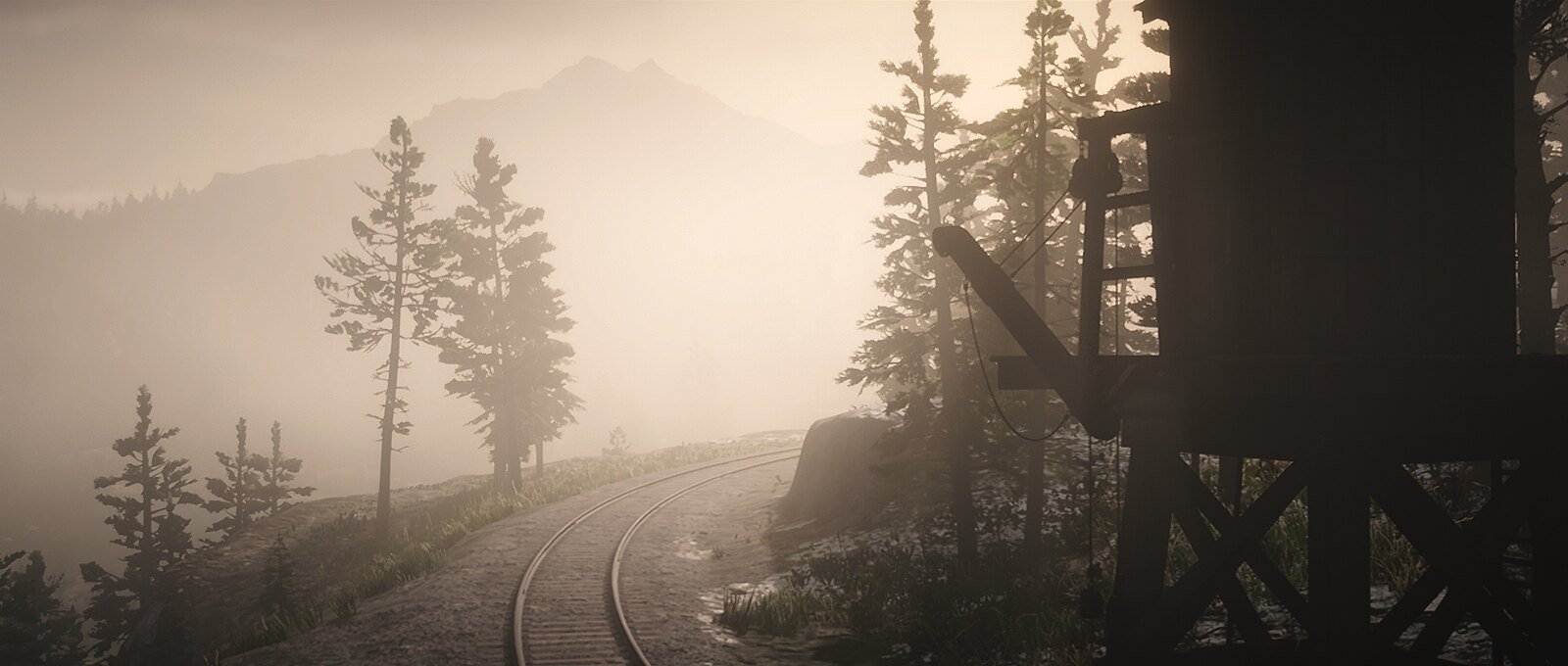A monochromatic outdoor photograph showcases a scene dominated by a curving railroad track that wraps over a hillside or mountainside, disappearing into a foggy, almost smoke-like atmosphere. On the right side, a distinctive barrel-shaped structure is built upon a wooden platform elevated by stilts. This structure is silhouetted against the cloudy backdrop, obscuring intricate details and rendering it dark. An arm protrudes from the side of the barrel-shaped structure, attached by a pulley system with cables designed to move the arm up and down. In the foreground, tall, slender evergreen trees rise up, their outlines stark against the hazy sky. The ground near the tracks is speckled with stone-colored aggregate, blending seamlessly with the overall forested ambiance. The peak of a distant mountain is barely visible through the dense clouds, adding a sense of depth and mystery to the scene. The entire image is imbued with a grayscale palette due to the poor lighting and overcast conditions, making it challenging to discern any vibrant colors but enhancing the atmospheric, almost ethereal quality of the landscape.